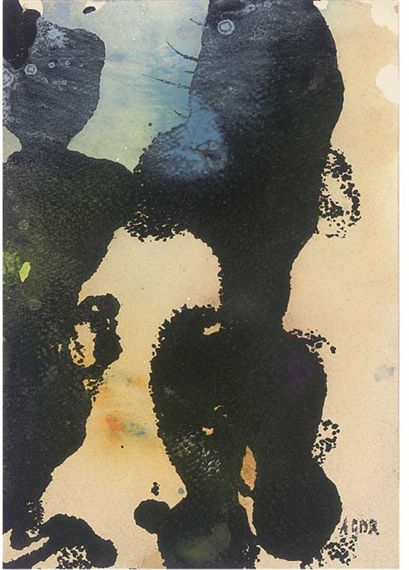The image is an abstract piece of art, vertically oriented and nearly twice as tall as it is wide. The background is predominantly yellow with light blue in the top left corner and hints of off-white or tan. The central focus consists of two large black ink blots that bear a rough resemblance to human figures. The first ink blot has a shape that suggests legs, hips, a midsection, and a wider top that could be interpreted as a head, though it's amorphous. This shape is connected on the left to a similar figure with a discernible head, neck, shoulders, torso, hips, and feet. Surrounding the main ink blots are various smaller dots and stains, including orange and blue between the figures, bluish stains at the top, and a greenish dot in the middle. At the bottom right, there is an unclarified marking resembling the stylized and incomplete letters "A-C-D-A." The overall appearance evokes the randomness and ambiguity of ink blots, with a slightly mirrored but asymmetric distribution.